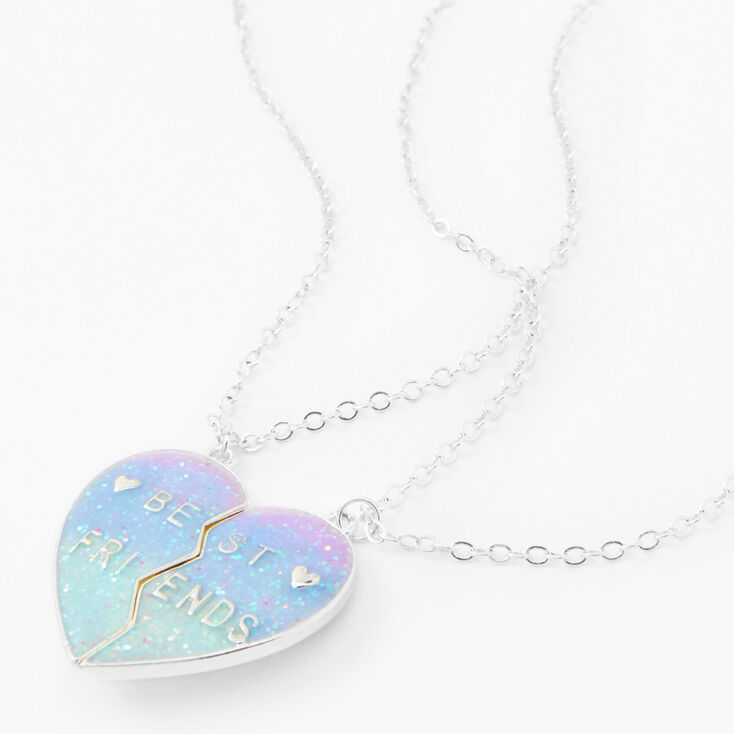This product image showcases a pair of sparkling friendship necklaces featuring heart-shaped pendants that split down the middle with a zigzag crack. Each silver-colored chain supports one half of the heart, and when placed together, the pendants form a complete heart with the phrase "Best Friends" written across it. The shimmering text "Best Friends" is silver and accompanied by small silver heart symbols next to the letters "B" and "T." The pendants display a mesmerizing gradient of pastel glitter colors, transitioning from purple at the top to blue in the middle, and finally to green at the bottom. Both the chains and the backs of the pendants possess a silver coating. The necklaces are displayed against a pristine white background, highlighting their delicate and enchanting design.